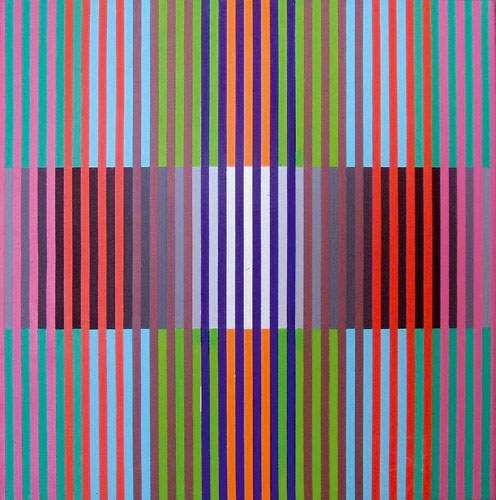The image is a vibrant and abstract piece of art that closely resembles the multicolored bars seen on a TV channel with no signal. It features a variety of contrasting colors, creating a dynamic and eye-catching composition. Vertical lines, starting pink on the left, transition through a spectrum of vibrant hues—reds, oranges, browns, blues, purples, and greens—before fading back to pink on the right. These lines stand in front of a multicolored background composed of teal, blue, green, and orange stripes, interspersed with gradients of green and blue to darker greens. Cutting through the middle of the image is a long silver bar with a white center, adding an additional layer of complexity to the composition. The interplay of these colors and shapes, with alternating lines and horizontal variations, generates a visually arresting depiction of contrast, light, and dark, seamlessly blending together in a harmonious visual symphony.